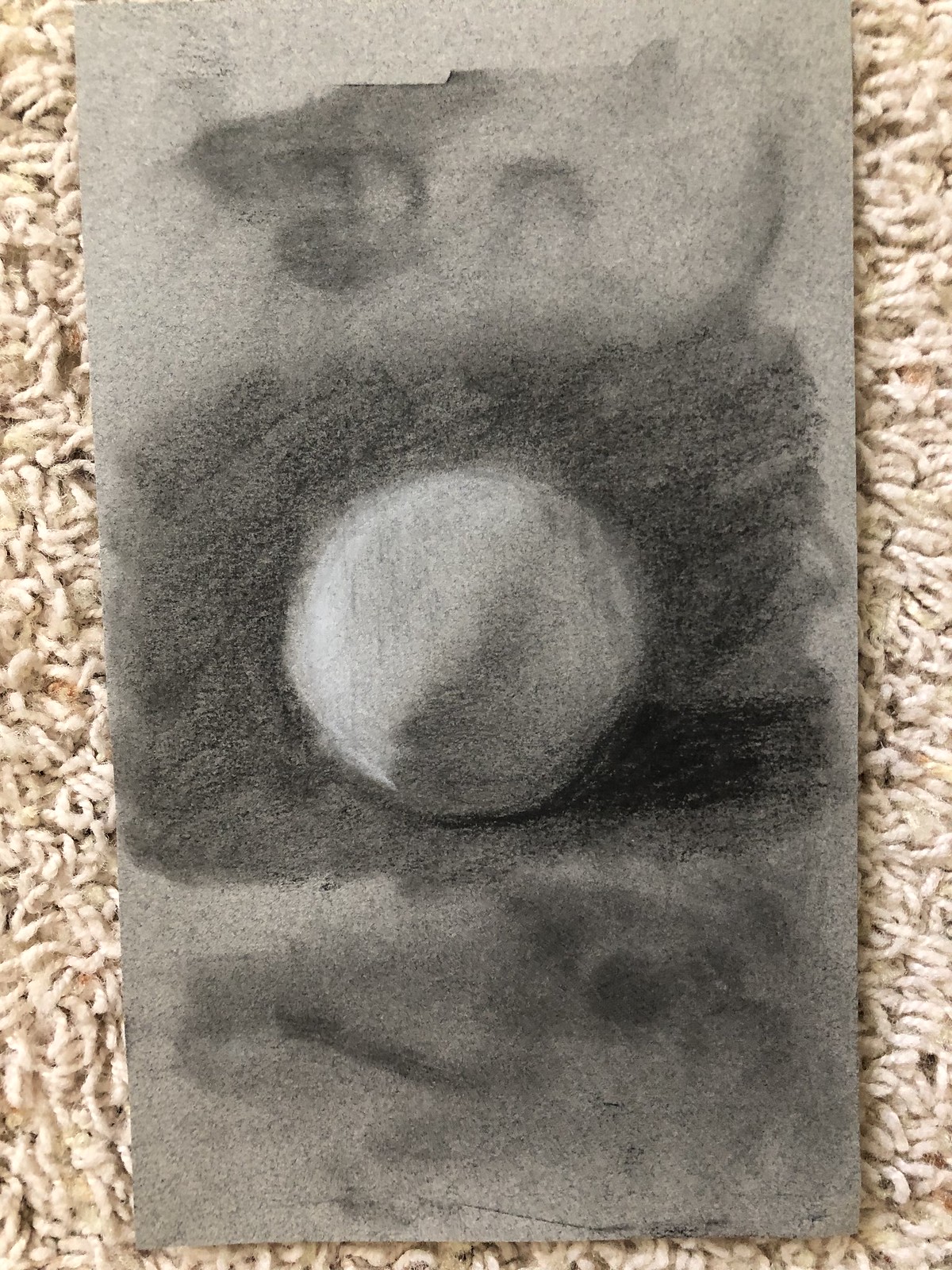This detailed drawing, rendered in shades of gray and black, is presented on a sheet of paper resting against a textured, shaggy tan surface. The composition features two dark gray, smoke-like forms flanking either side, creating a dynamic frame for the central figure. At the core of the drawing is a shape reminiscent of a moon, with its upper portion in an off-white hue and its lower section in a deeper gray, contributing to a striking contrast. The background behind the central moon shape is filled with a rich black, adding depth and intensity to the artwork. The image bears a unique, almost distressed texture, akin to the effect achieved when water spills on paper, giving it a partially 'bleeding' and slightly damaged appearance. Despite this, the quality of the artwork remains impressive, adding to the overall aesthetic and emotional impact of the piece.